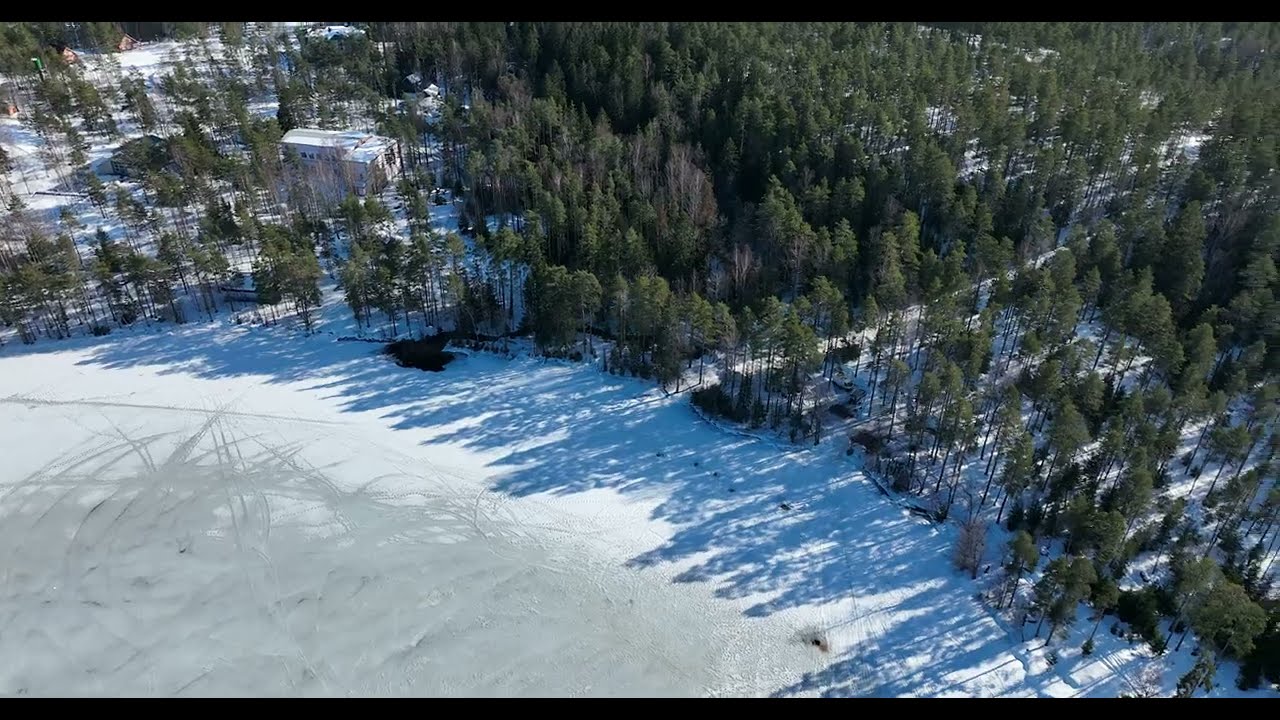This aerial photograph captures a serene winter landscape dominated by a dense forest interspersed with patches of snow-covered ground. Towards the bottom of the image, a frozen lake or pond is visible, with tracks suggesting recent activity, possibly ice skating, on its surface. The snow appears gray and dark in the long shadows cast by the trees, a mix of pine and leafy varieties, and the ice is tinged a gray-green hue beneath the snow. To the left side of the photo, in the distance among the trees, several buildings and houses can be seen, standing out against the natural backdrop. The absence of the sky and any visible human activity adds to the tranquil and undisturbed quality of the scene. The composition is primarily a blend of white snow and green forest, presenting a striking contrast in this cold, late-day snowscape.